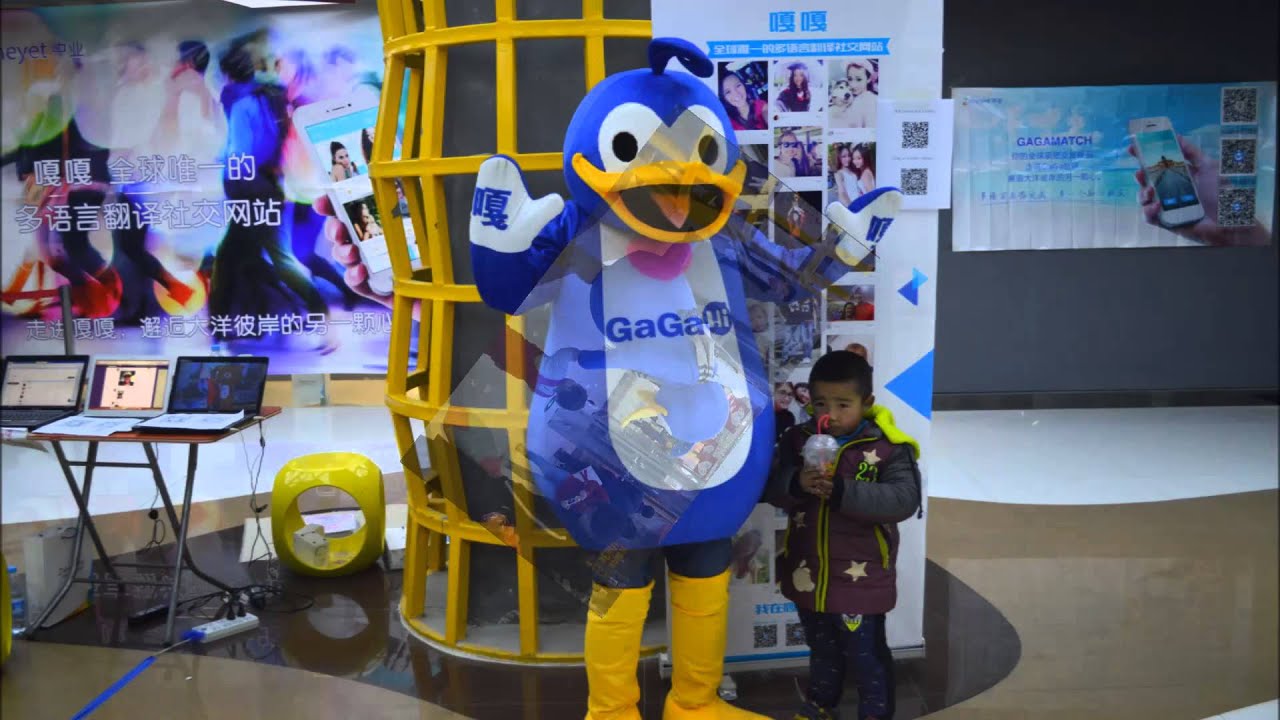The photograph captures a lively indoor event or convention with a colorful environment. Dominating the foreground is a large, blue cartoonish penguin mascot, actually a person inside a suit. The mascot stands center-frame, featuring a teardrop-shaped torso with a blue body, white stomach, and yellow beak. The stomach bears blue text that reads "Ga Ga," and the hands, ending in mitts, display Asian characters on white palms. The mascot's head, with a playful swoop of hair feathers, features large white eyes with black pupils and a wide, cheerful yellow beak.

Next to the mascot is a small, upset-looking child who appears to be Asian, wearing a purple and green jacket adorned with white stars and blue jeans. The child clutches a drink with a red straw, adding a touch of everyday life to the scene.

In the background, the setting bustles with activity, including various posters and signs in an Asian language. To the left, atop a brown portable desk, three laptops sit open amidst a tangle of electrical cords. On the wall, abstract imagery and Asian text highlight the diverse, multilingual essence of the event. The wall text proclaims, "Gaga is the only multilingual translation social network site in the world" and "across the ocean of Gaga," emphasizing the global connectivity theme. Additionally, a metal tubular structure with yellow bars stands directly behind the mascot and child, adding a dynamic industrial element to the scene. The floor beneath them appears to be tiled in multiple colors, completing the vibrant, bustling atmosphere of the photographed event.